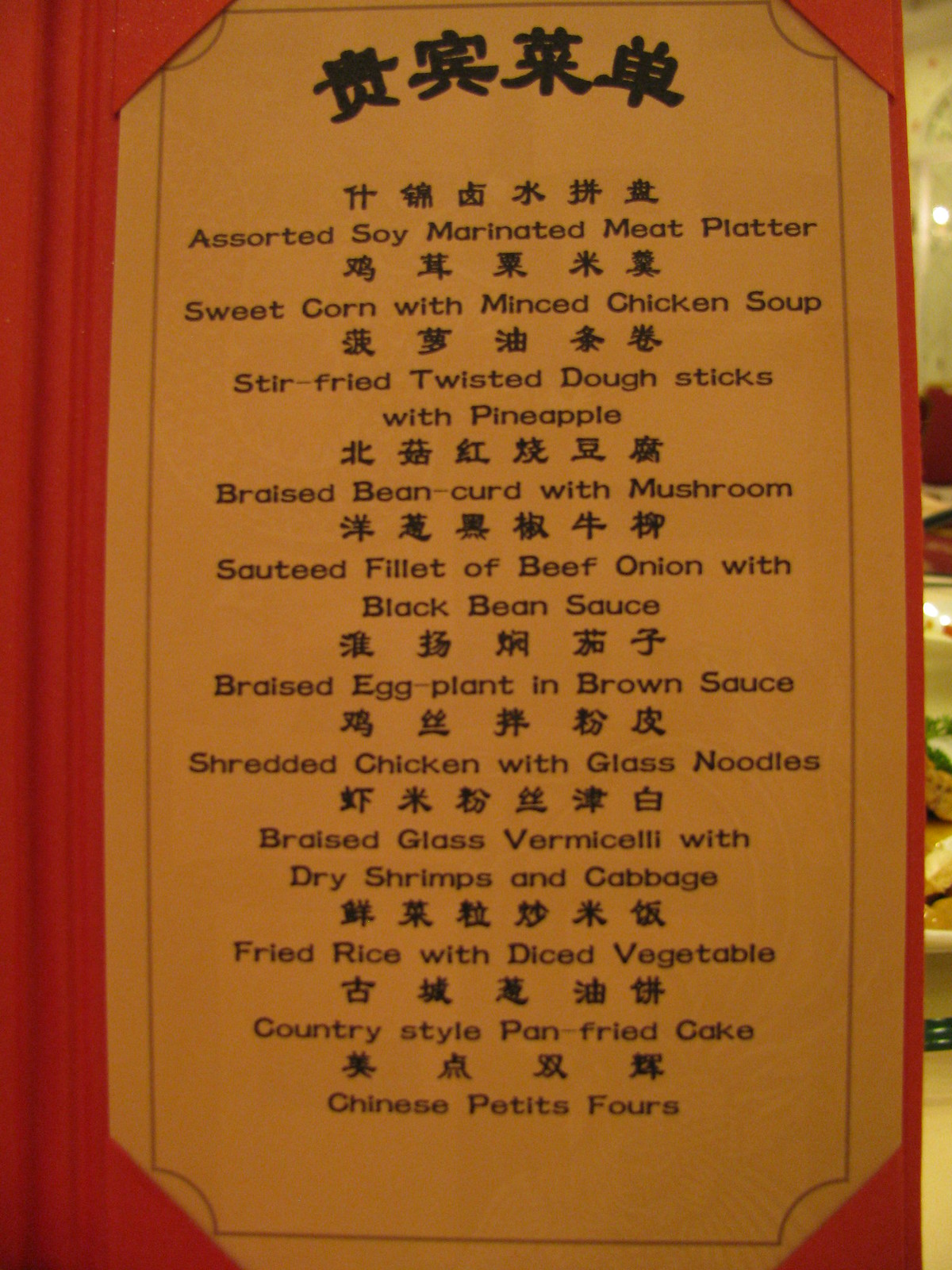The photograph showcases a detailed image of a menu set against the backdrop of a restaurant interior. The menu insert, made of brown paper, is securely held within a red fabric menu shell, which features small triangular holders at each corner to keep the insert in place. The top section of the menu is adorned with Chinese characters, which provide an authentic touch to the menu items listed below each set of characters in English. The menu includes a variety of dishes such as an assorted soy-marinated meat platter, sweet corn with minced chicken soup, stir-fried twisted dough sticks with pineapple, braised bean curd with mushroom, sautéed filet of beef with onion and black bean sauce, braised eggplant in brown sauce, shredded chicken with glass noodles, braised glass vermicelli with dried shrimps and cabbage, fried rice with diced vegetables, country-style pan-fried cake, and Chinese petit fours. To the right edge of the photograph, there is a glimpse of the restaurant's interior, hinting at the ambiance and setting where this menu is offered.